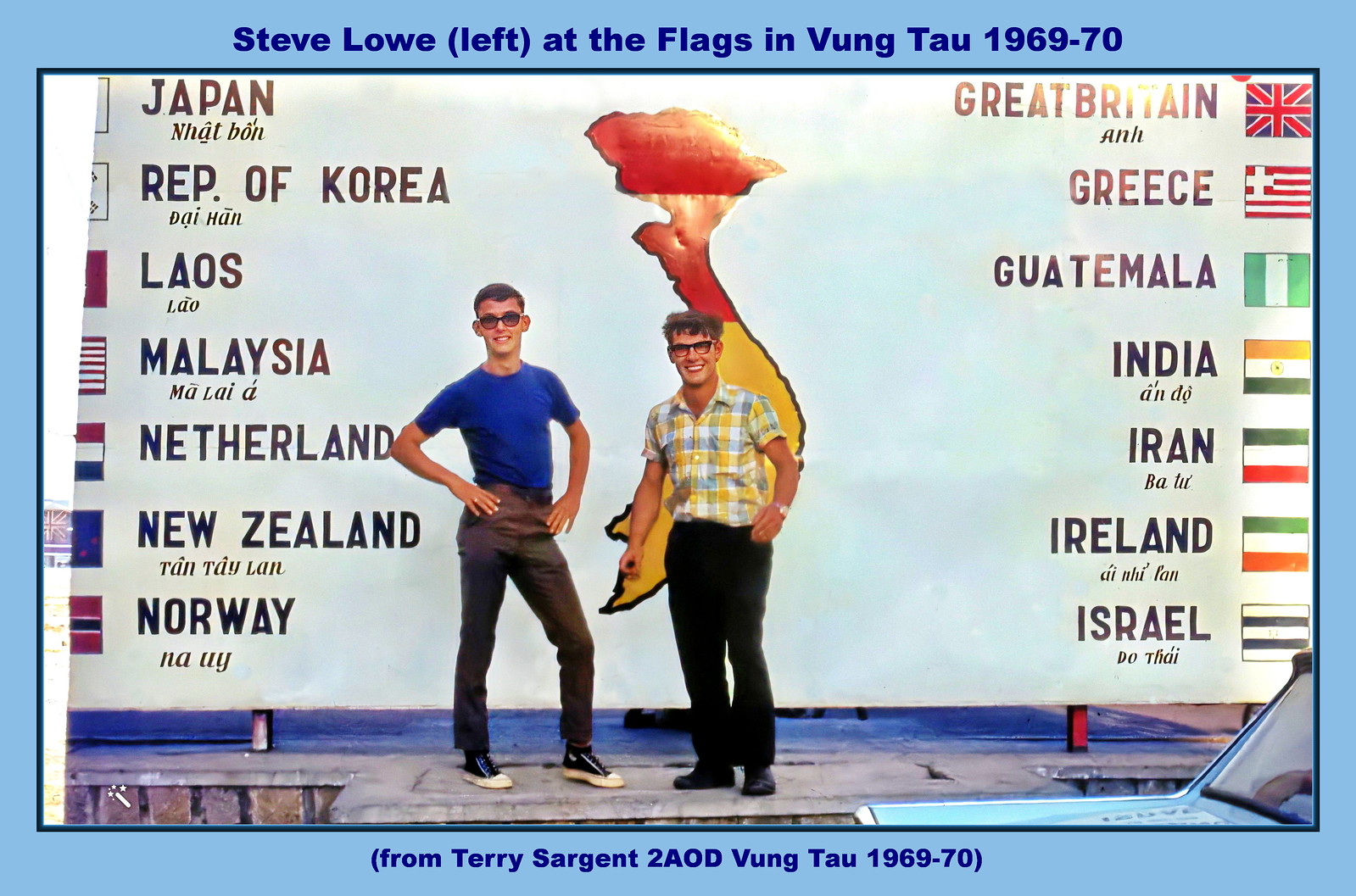This color photograph, framed with a blue border and blue text at the top and bottom, captures a nostalgic moment from Vung Tau, 1969-70. At the top of the image, the text reads: "Steve Lowe (left) at the flags in Vung Tau 1969-70," while the bottom text states, "(from Terry Sargent to AOD Vung Tau 1969-70)." The photograph features two young Caucasian men wearing glasses, standing in front of a large billboard listing countries and their flags. The man on the left stands near the center, wearing a blue shirt, brown pants, and black and white Chuck Taylor shoes, with his hands on his hips. To his right is a slightly shorter man in a white, yellow, and gray plaid shirt with black pants and black shoes, one hand in his pocket. The billboard behind them displays the names and flags of various countries: Japan, Republic of Korea, Laos, Malaysia, Netherlands, New Zealand, Norway on the left side, and Great Britain, Greece, Guatemala, India, Iran, Ireland, Israel on the right side. Additionally, there is an edge of a blue vehicle visible at the lower right corner of the image, suggesting this stage might have been set for a larger event or gathering. Both men are smiling, adding a personal touch to this historical snapshot.